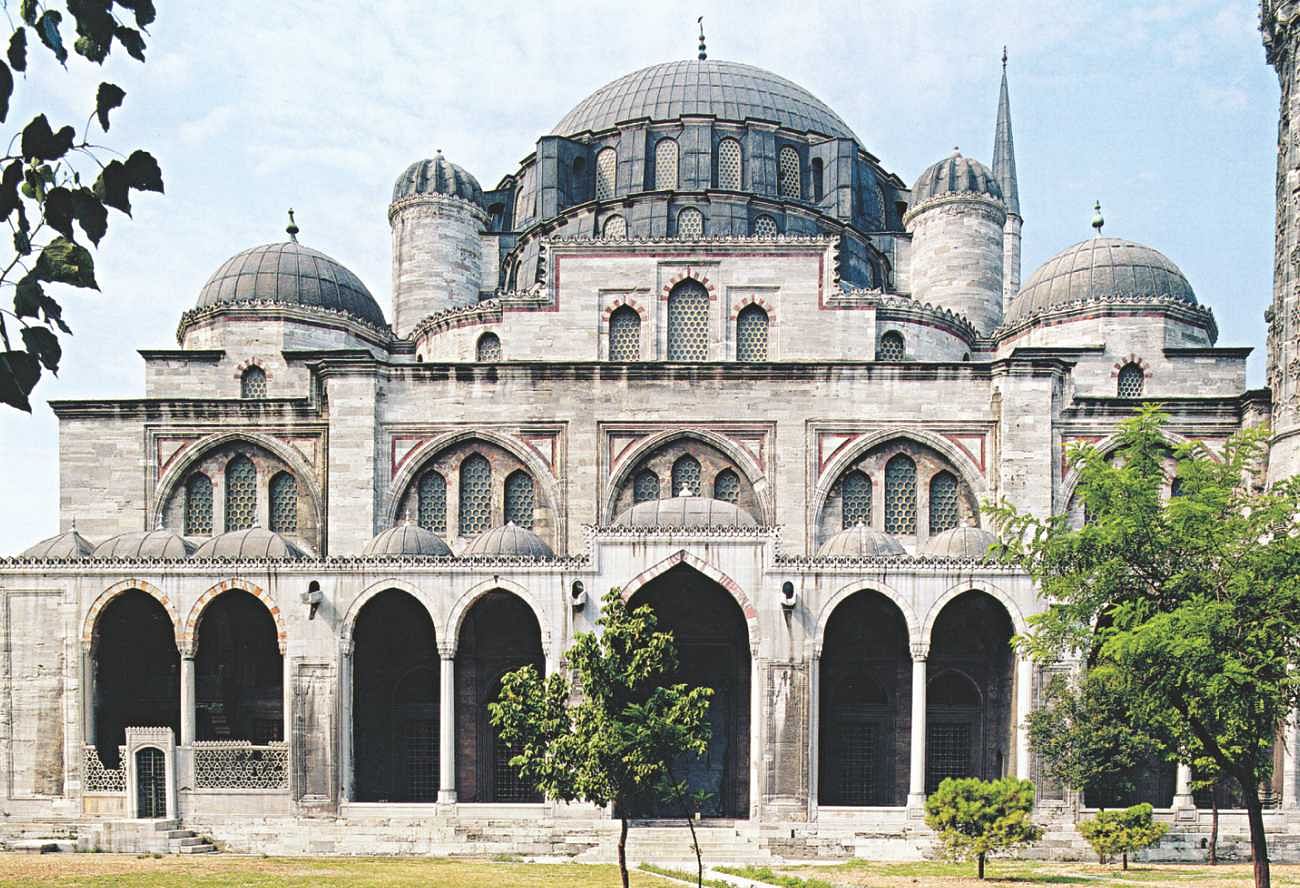The image captures an old, ornate building resembling a grand Middle-Eastern mosque, palace, or cathedral with architectural elements that conjure thoughts of both Russian influences and medieval times. The structure prominently features a series of domes: one large central dome, two medium-sized domes on either side, and smaller ones nestled between these central and side domes atop slender towers. The building, constructed primarily from white marble and light beige material, boasts multiple archways and arched windows, which are small and slender, grouped in threes above each section. The topmost dome is gray, contrasting with the lighter colors of the building. 

The entrance is marked by several pillars and multiple archways, with a larger central opening flanked by pairs of smaller arches. The scene is set against a cloud-filled blue sky, adding to the majestic aura of the structure. The foreground is dotted with a few trees and shrubs, including a small tree directly in front of the main door, and an additional tree to the right. The left upper corner features some green leaves, possibly from an off-frame tree. The overall impression is that of a slightly weathered yet grand establishment with a blend of influences, radiating historic and cultural richness.